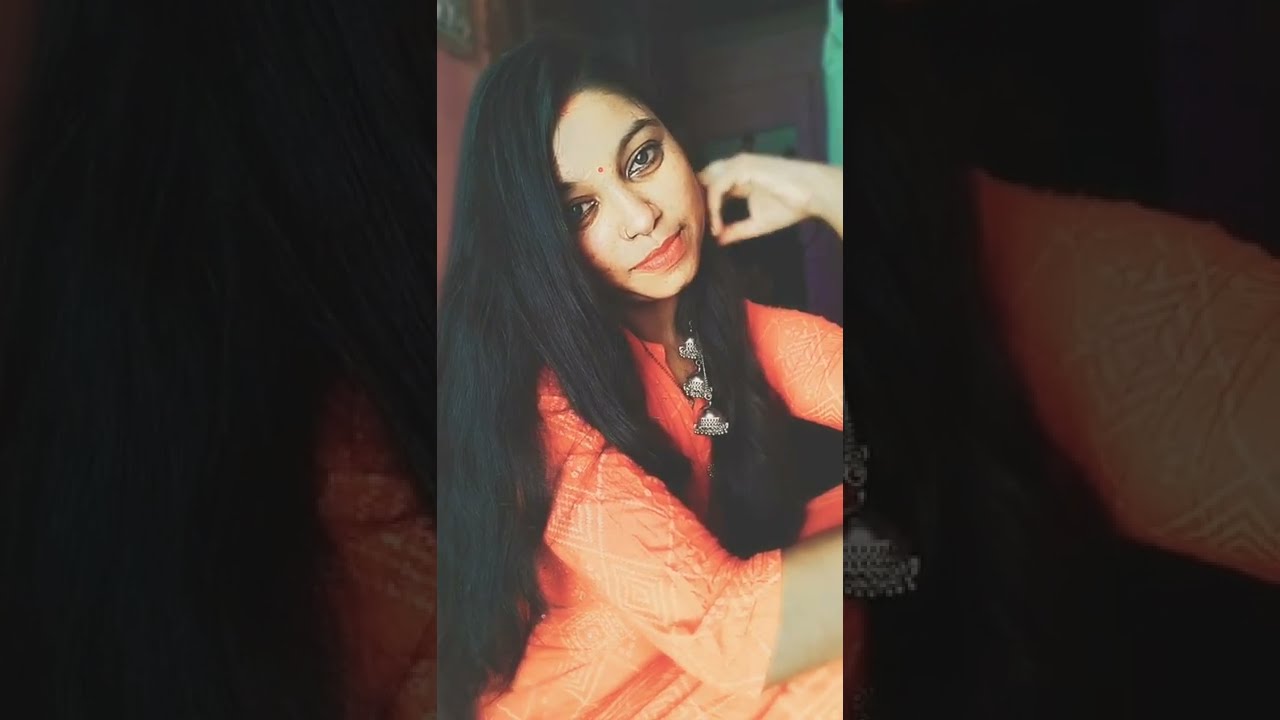This is a detailed photograph of a young woman, likely of Indian or Pakistani descent, whose image is artistically presented. The composition features a central photograph of the woman, superimposed over an enlarged, darkened version of the same image that serves as the background. The woman captivates attention with her long, straight black hair cascading past her shoulders, framing her face as she stares at the camera with dark, expressive eyes and a slight smile.

She is dressed in an orange elbow-length tunic-style dress, adorned with a diamond pattern that includes smaller diamonds descending in size toward the center. Intricately detailed, the dress also features an Indian or Aztec type design with a light faded line. Her accessory choice stands out; she wears a prominent silver necklace or earrings with at least three distinct tiered pendants, adding a touch of elegance, although the low resolution makes the specific details of the pendants indistinct.

In the photograph, the woman strikes a thoughtful pose, her right shoulder angled closer to the camera. Her head tilts slightly downward, her hand gently resting on her chin, giving a contemplative air to her demeanor. The use of the enlarged and darkened version of her photograph as the left and right backdrop contrasts beautifully with the vivid colors of her clothing and features, highlighting her central presence and adding depth to the image.